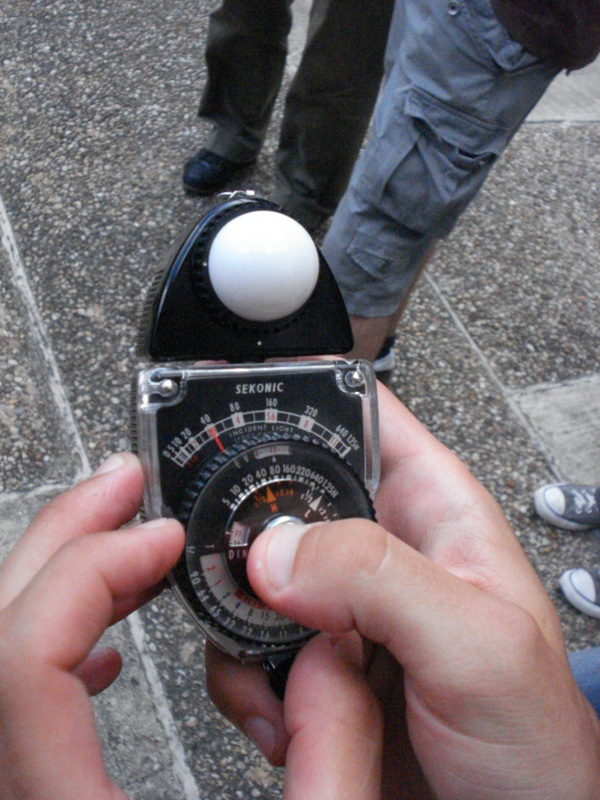In the photograph, a pair of hands are carefully holding an intriguing vintage device labeled "C conic." The gadget, adorned with various dials and indicators, appears to be an old-fashioned light meter used for photography, as suggested by the inscription "incident light." Its design features a striking white dome at the top, contrasted by a black base and encased in a sleek silver frame. The individual is seen actively adjusting the dials on the device.

In the background, a sidewalk is partially visible where several people are walking. One person is dressed in grey cargo pants paired with black sneakers. Another individual is sporting brown pants and black hiking boots or high shoes. A third person is wearing tennis shoes, although their legs are not visible in the frame. Additionally, there is a fleeting glimpse of someone in blue jeans, though the image captures only a minimal portion of this attire. The scene provides an engaging mix of vintage technology and everyday street activity.